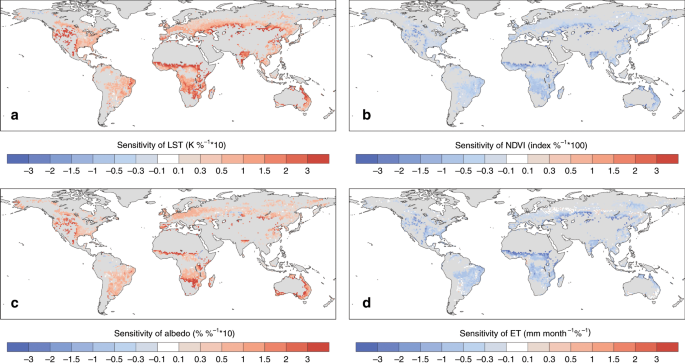The image consists of four detailed maps arranged in two rows and two columns, each labeled A, B, C, and D. Every map portrays a flat representation of the globe with gray continents and white oceans. Map A, in the upper left corner, features red markings on the continents and includes the text "sensitivity of LST (k%^-1)*10" with a color scale ranging from -3 to 3. Map B, positioned to the right of Map A, shows blue markings and reads "sensitivity of NDVI (100%^-1)" alongside a similar color spectrum from -3 to 3. Map C, found in the lower left, also displays red markings and is labeled with "sensitivity of albedo (percentage^-1)" and the color scale from -3 to 3. Finally, Map D, in the lower right corner, is marked with blue and includes the text "sensitivity of ET (mm/month^-1)" with the same color gauge from -3 to 3. All the maps share a consistent format with a gray landmass, white water bodies, and a color spectrum bar beneath each map to interpret the data ranges. There are no people in the image, and the primary focus remains on the geographical data represented.